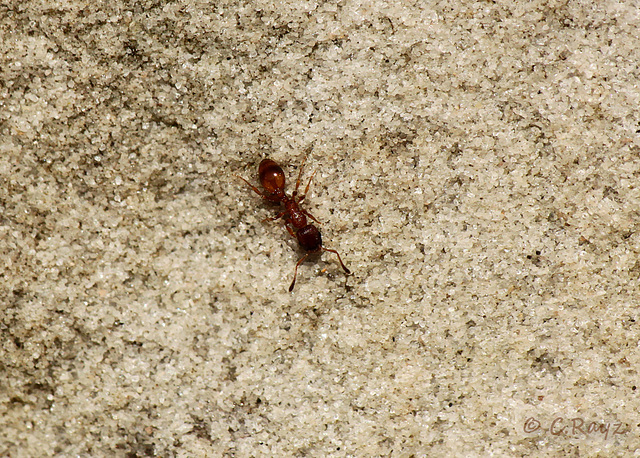This photograph showcases a close-up, detailed view of a red ant standing on a textured, grainy surface of sand. The sand displays various shades, predominantly off-white with some tan, brown, and black kernels. In the center of the image, the red ant is prominently featured, facing downward and slightly to the right. The ant's body consists of three distinct segments: a round, dark red head with two antennae, a long and thin oval thorax, and a bulbous, egg-shaped abdomen. The ant's six thin legs extend outward from its body, positioned in different directions. The sand beneath it appears finer on the right side and darker on the left, adding depth to the overall composition. In the bottom right corner, there is a copyright mark "CZ."